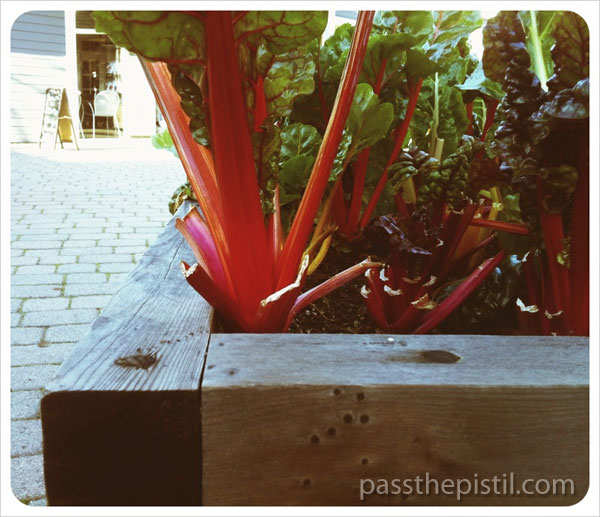This image shows a detailed close-up of a corner of a raised wooden planter filled with various plants, including prominently featured large, red-stemmed rhubarb plants with green and purple leaves. The planter itself is constructed from wooden planks and is filled with rich soil. The setting appears to be outdoors, perhaps in a public area or the back area of a business. In the background, to the left, there is a stone-covered ground, a building with its door open, a white chair positioned in front of the doorway, and a chalk sandwich board sign. Additionally, gray text in the bottom right corner of the image reads "passthepistol.com." This notable scene is encompassed within a square border, capturing both the lush vegetation and elements of the surrounding environment.